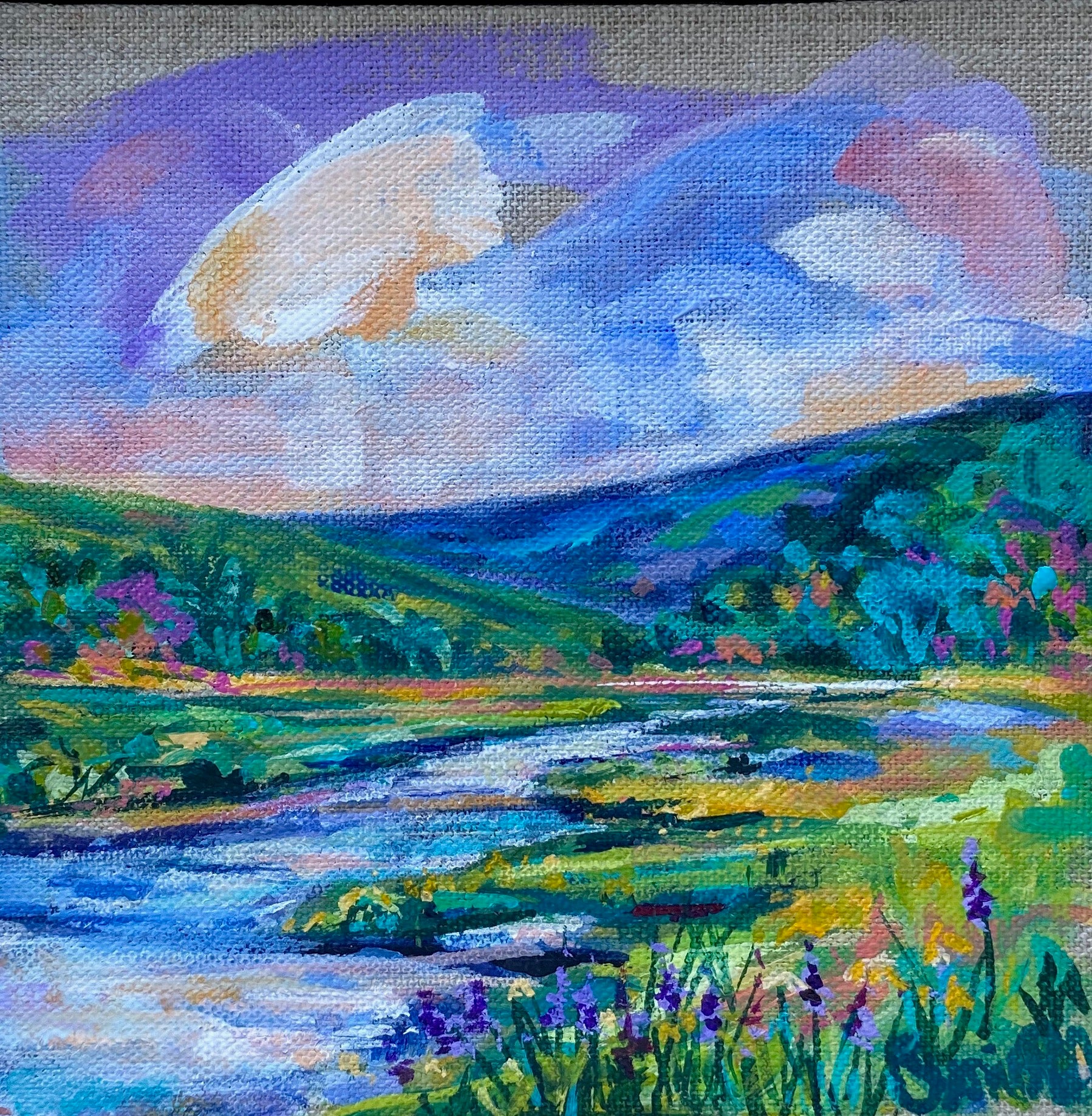This image showcases a vivid and colorful painting on a gray canvas, likely created using acrylics. The scene depicts a tranquil river with clear blue water reflecting a vibrant sunset in the sky above. The sky is a mesmerizing blend of colors, including blue, yellow, orange, pink, red, and white clouds. In the background, there are majestic mountains or hills shaded in green with patches of yellow. The foreground is rich with a variety of colorful foliage: green grass peppered with flowers in shades of purple, pink, magenta, and yellow. These include distinctive purple lupine flowers. The left side of the painting features a green hill brightly accented with hues of purple, pink, and light orange, while the right side displays fields with tones of aqua blue, dark green, and pink. The uppermost part of the painting has a small section of the raw gray canvas visible, adding a unique touch to this serene and vividly detailed nature scene.